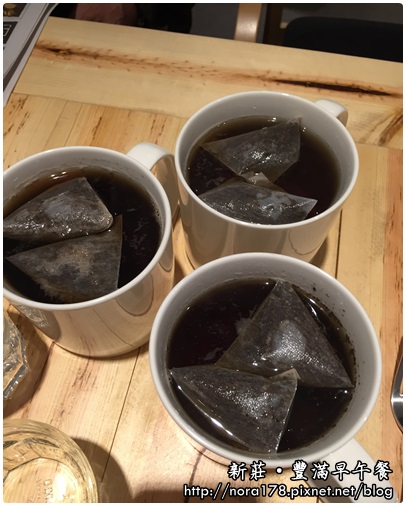In this photograph, we see three white ceramic coffee cups filled with what is presumably black tea, evidenced by the teabags floating on the top surface of each cup. Each teabag contains two triangular bags, fully submerged and bulging, indicating they are well-steeped. The cups rest on a light brown, slightly stained tabletop with visible knots and lines. In the bottom right-hand corner of the image, there are Mandarin characters above a website link, http://nora178.pixnet.net/. Additionally, the bottom left-hand corner of the image shows an empty glass serving cup. A partially visible chair and possibly clear coasters or covers are also present in the background.